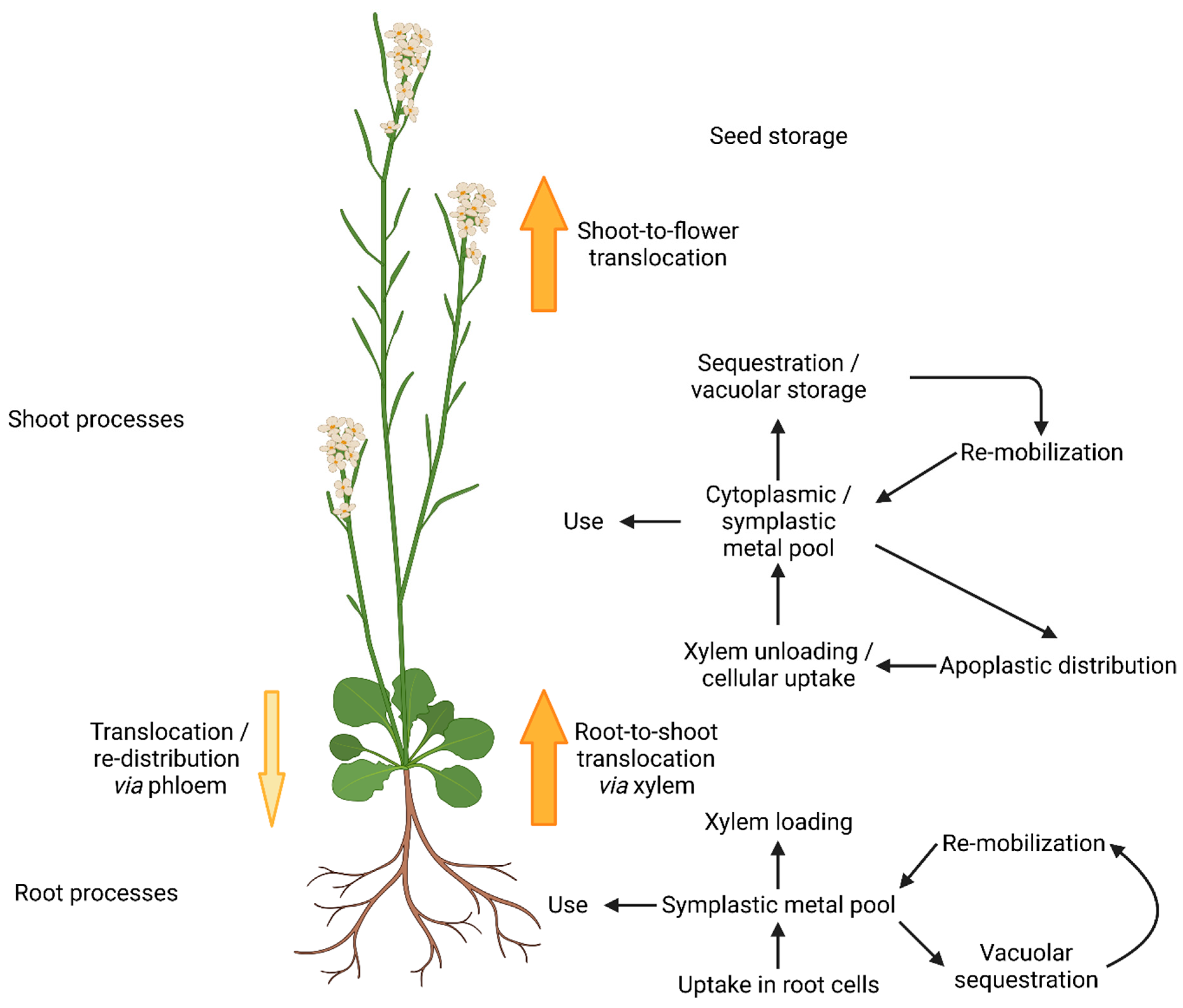The image is a detailed scientific drawing of an entire plant system, showcasing both the shoot and root processes. The artistic rendering depicts tall, brown stems extending upwards with small green leaves emerging, and white flowers, each with yellow cores, adorning the tops of the stems. The base features the root system, from which the plant's growth begins. The diagram includes numerous annotations, pointing to various parts of the plant, explaining processes such as the "shoot process" and "root process."

Key labels and arrows describe detailed biological activities, including "shoot to flower translocation," "root to shoot translocation via xylem," "cytoplasmic symplastic metal pool," "cellular uptake," "apoplastic redistribution," "vacuolar sequestration," "xylem loading," and "remobilization." The image also emphasizes "seed storage," highlighting the life cycle completion as seeds fall to the ground, initiating the growth of a new root system.